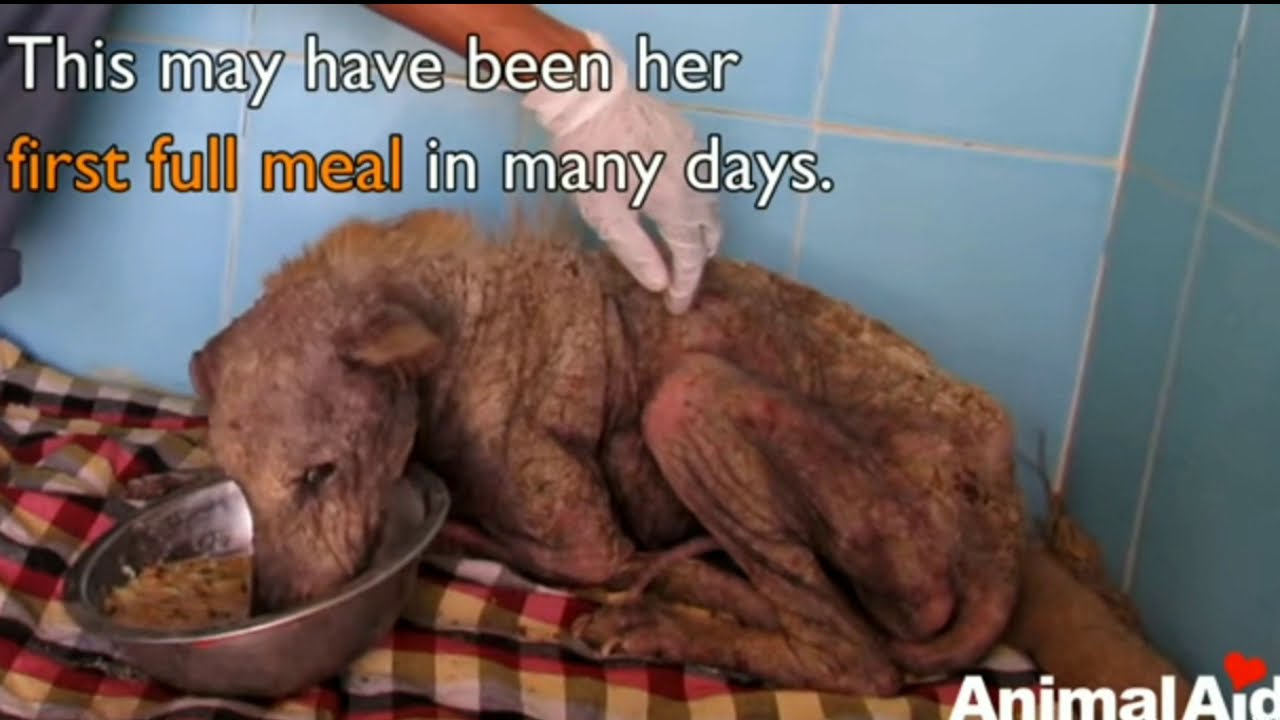The image depicts an emaciated, large dog in a severely neglected condition, almost skeletal with patches of red, irritated skin and missing fur. The dog is sprawled out on a checkered blanket that features red, white, black, and yellow squares. It is centered in the image, with its head buried in a metal bowl, possibly eating what might be its first full meal in many days. The animal's back legs are splayed outward, highlighting the wrinkles in its skin. A hand wearing a white latex glove extends into the frame from the top, gently touching the dog's back, possibly indicating a medical examination or some form of comfort. The background consists of light blue tiles with white grout. There is text on the image stating, "this may have been her first full meal in many days," with "first full meal" highlighted in orange. Additionally, the bottom right corner of the image features the text "animal aid," adorned with a red heart atop the second 'i'. The overall scene is somber, accentuated by the dog's dire state and the clinical setting.